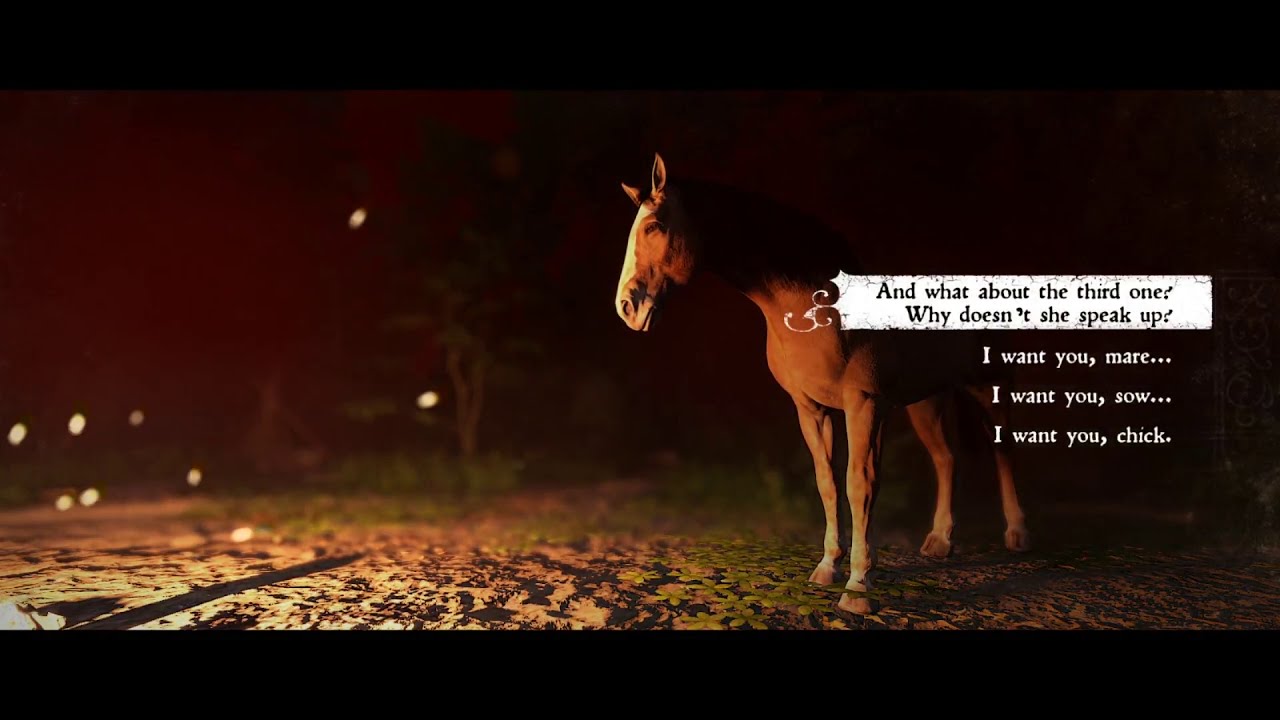The scene depicts a dark, nighttime atmosphere enveloped in a muted reddish-brown sky, with a few silhouettes of trees visible in the background. The ground is scattered with leaves, hinting at an autumn setting, and there is a faint hint of a road beneath the foliage. Dominating the right side of the picture is a solemn-looking animal, possibly a donkey or horse, with a distinctive white blaze down its brown face, adding a touch of contrast to the otherwise shadowy environment. The widescreen format of the image is evident through the black bars at the top and bottom, creating a cinematic effect. Superimposed over the animal is a white rectangular box containing black text that reads: "And what about the third one? Why doesn’t she speak up?" Below this, another line of text elaborates: "I want you, mayor... I want you, sow... I want you, chick." The artful juxtaposition of the animal’s contemplative gaze and the enigmatic textual elements culminate in a poignant visual narrative.